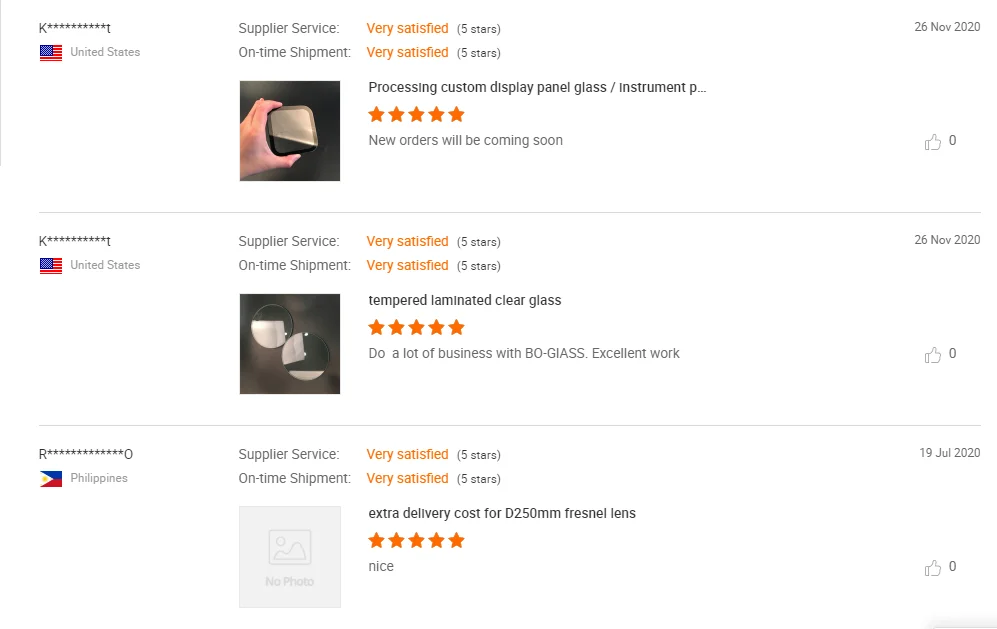**Image Description:**

This image displays a section of a retail website showcasing customer reviews and ratings for various products and services.

1. **First Review Section (Left)**
   - **Reviewer:** K****T from the United States (with the U.S. flag underneath their initials).
   - **Supplier Service:** Very Satisfied (5 stars).
   - **On-Time Shipment:** Very Satisfied (5 stars).
   - **Picture:** A white hand holding a square object.
   - **Product/Service Detail:** "Processing custom display panel glass/instrument."
   - **Customer Feedback:** "New orders will be coming soon."

2. **Second Review Section (Center)**
   - **Reviewer:** K****T from the United States (with the U.S. flag underneath their initials).
   - **Supplier Service:** Very Satisfied (5 stars).
   - **On-Time Shipment:** Very Satisfied (5 stars).
   - **Picture:** Two round discs, presumably made of glass.
   - **Product/Service Detail:** "Tempered laminated clear glass."
   - **Customer Feedback:** "Do a lot of business with Bioglass, excellent work."

3. **Third Review Section (Right)**
   - **Reviewer:** R****O from the Philippines (with the Filipino flag next to their initials).
   - **Supplier Service:** Very Satisfied (5 stars).
   - **On-Time Shipment:** Very Satisfied (5 stars).
   - **Picture:** No photo provided.
   - **Product/Service Detail:** "Extra delivery cost for D250 millimeter Fresnel lens."
   - **Customer Feedback:** "Nice."

Each review includes detailed satisfaction ratings and feedback, complemented by relevant product images where available. The reviews reflect high customer satisfaction with supplier service and on-time shipments.